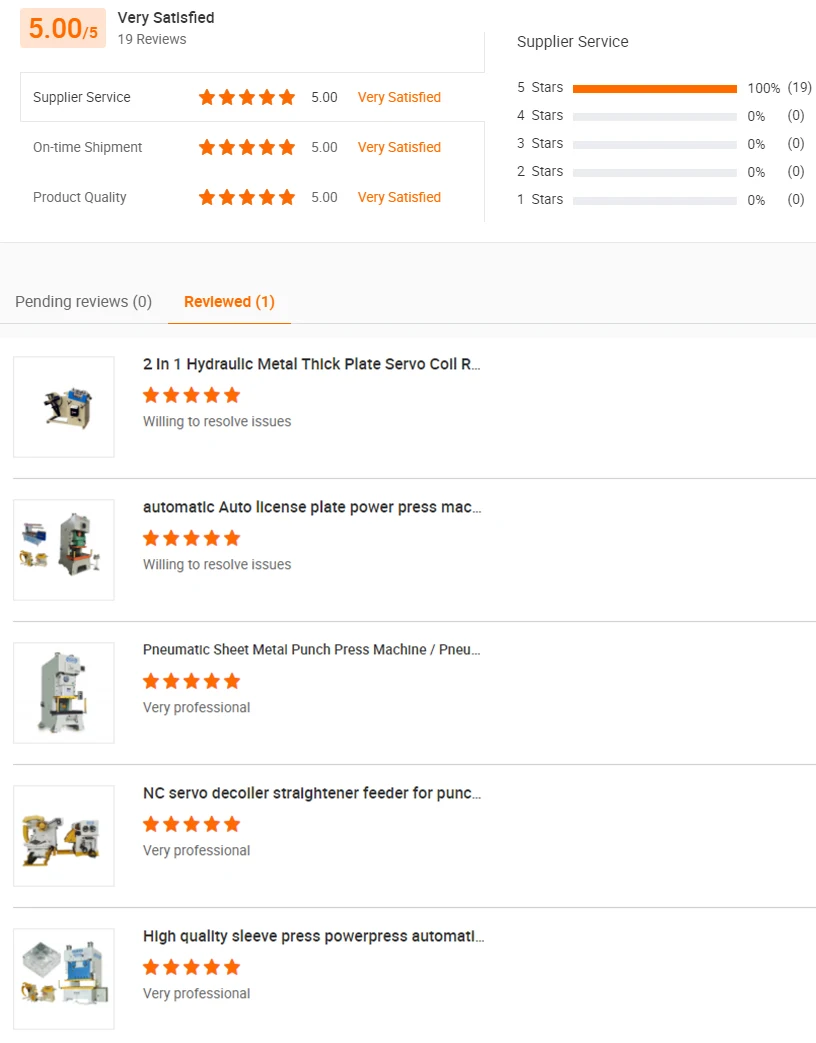**Detailed Descriptive Caption:**

The image features a predominantly white background with a series of ratings and reviews encapsulated within a prominent pink box at the top. Inside this box, the ratings are detailed as follows:

- **Overall Supplier Service:** Rated five stars (5.00) with "very satisfied" indicated by 19 reviews.
- **On-Time Shipment:** Also rated five stars (5.00) with feedback marked as "very satisfied."
- **Product Quality:** ACHIEVING a perfect five stars (5.00) with reviewers "very satisfied."

Below these top-tier ratings, there are sections detailing specific reviews and pending issues for various machinery items:

1. **Hydraulic Metal Thick Plates of Coal:** Rated five stars, but there are pending reviews or issues awaiting resolution.
2. **Automatic Auto License Plate Power Press Machine:** Mentioned with a five-star rating, but similarly awaiting resolution.
3. **Pneumatic Sheet Metal Punch Press Machine (New):** Rated five stars, described as "very professional."
4. **NC Servo Decoiler Straightener Feeder for POON:** Rated five stars, highlighted as "very professional."
5. **High-Quality Sleep Press Power Press Automatic:** Additionally rated five stars, acclaimed for being "very professional."

The caption ends by noting the supplier service is rated five stars with a 100% satisfaction rate. Beyond this pink box and detailed ratings, there is a noticeable expanse of empty white space.